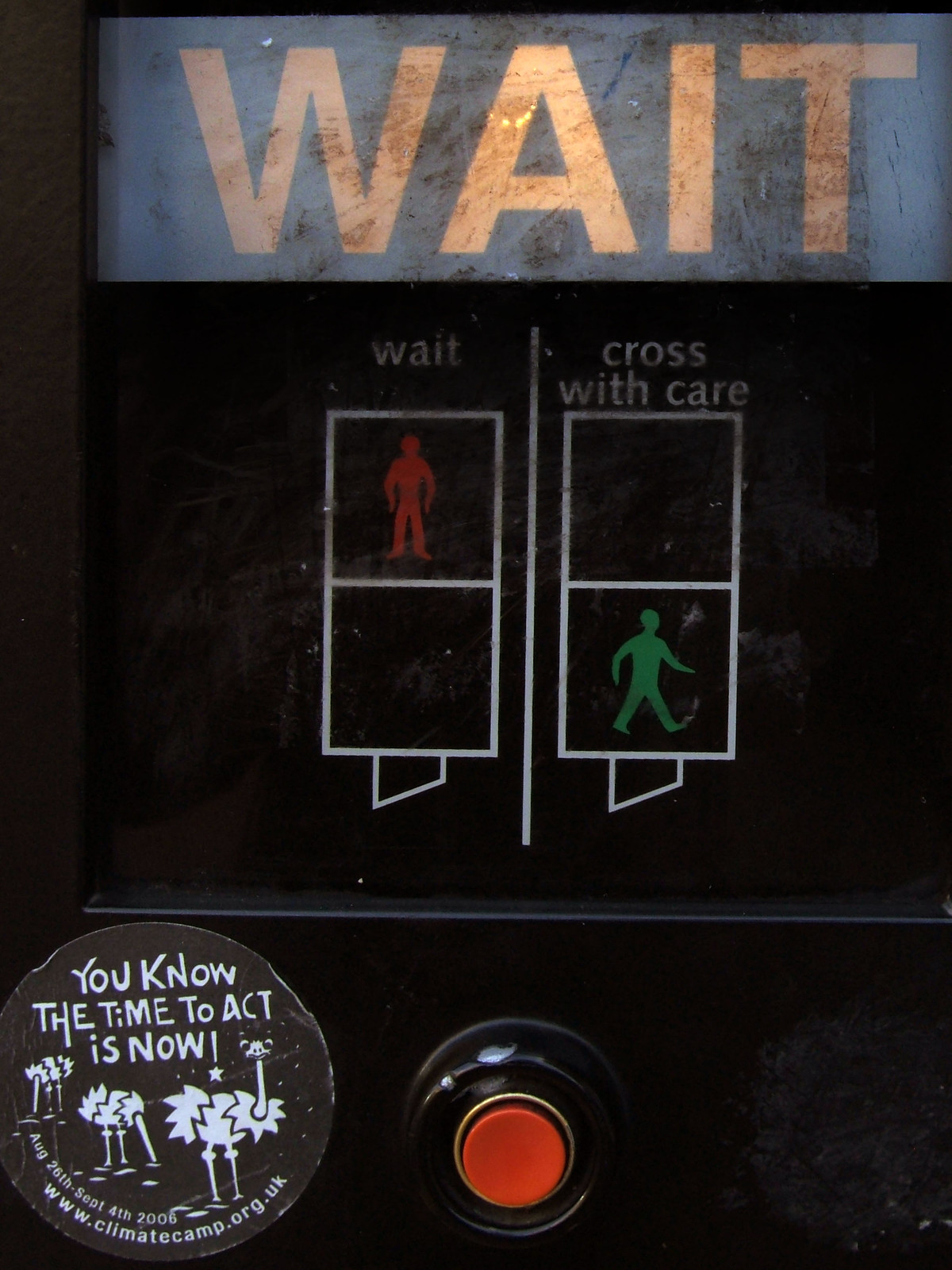The image is a vertical rectangular close-up of a traffic control device typically found at a crosswalk. At the top of the device is a slightly dirty, blue backlit sign that reads "WAIT" in white text. Below this, the panel is divided into two sections with visual indicators: on the left side, a red figure standing still next to the word "WAIT," and on the right side, a green figure walking next to the words "CROSS WITH CARE." The purpose of these indicators is to show pedestrians what to look for on the accompanying traffic signals.

At the bottom center of the image is a large red button designed for pedestrians to press when they want to signal a change in the crosswalk light. To the left of this red button is a round sticker, which adds a unique touch to the device. The sticker features three ostriches, with two of them having their heads in the sand, and it carries a message in white letters: "You know the time to act is now." The sticker includes information about a climate change organization, promoting awareness and action. The colors present in this image include black, red, white, green, tan, and blue. The overall setting suggests an urban environment near an intersection.